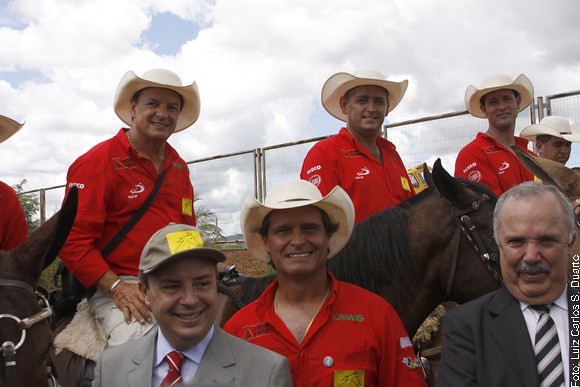This color photograph, taken outdoors during the daytime, captures a group of eight men, five on horseback and three standing in front of them, against a backdrop of a metal fence and a sky dotted with fluffy white clouds. The image is in landscape orientation, wider than it is tall. The men on horseback are wearing matching outfits consisting of red long-sleeved shirts and cream-colored cowboy hats, each featuring a small yellow square with a horse head emblem. 

The three men in front, standing from the upper chest up, are all facing the viewer. On the right is an older man with a receding hairline, gray hair, and a gray mustache, dressed in a gray suit and tie. In the center stands a man in a red polo shirt and a white cowboy hat. To the left is a shorter man in a light gray suit, white shirt, and red tie, sporting a light gray baseball cap with a similar yellow square emblem. 

The four men on horseback, positioned behind these three, are all of Caucasian descent and similarly attired in red shirts and white cowboy hats. The visible portions of the horses indicate they are brown. Flanking the scene on the edges, partially cut off, are additional figures in similar hats. The overall composition showcases a cohesive, representational realism style.